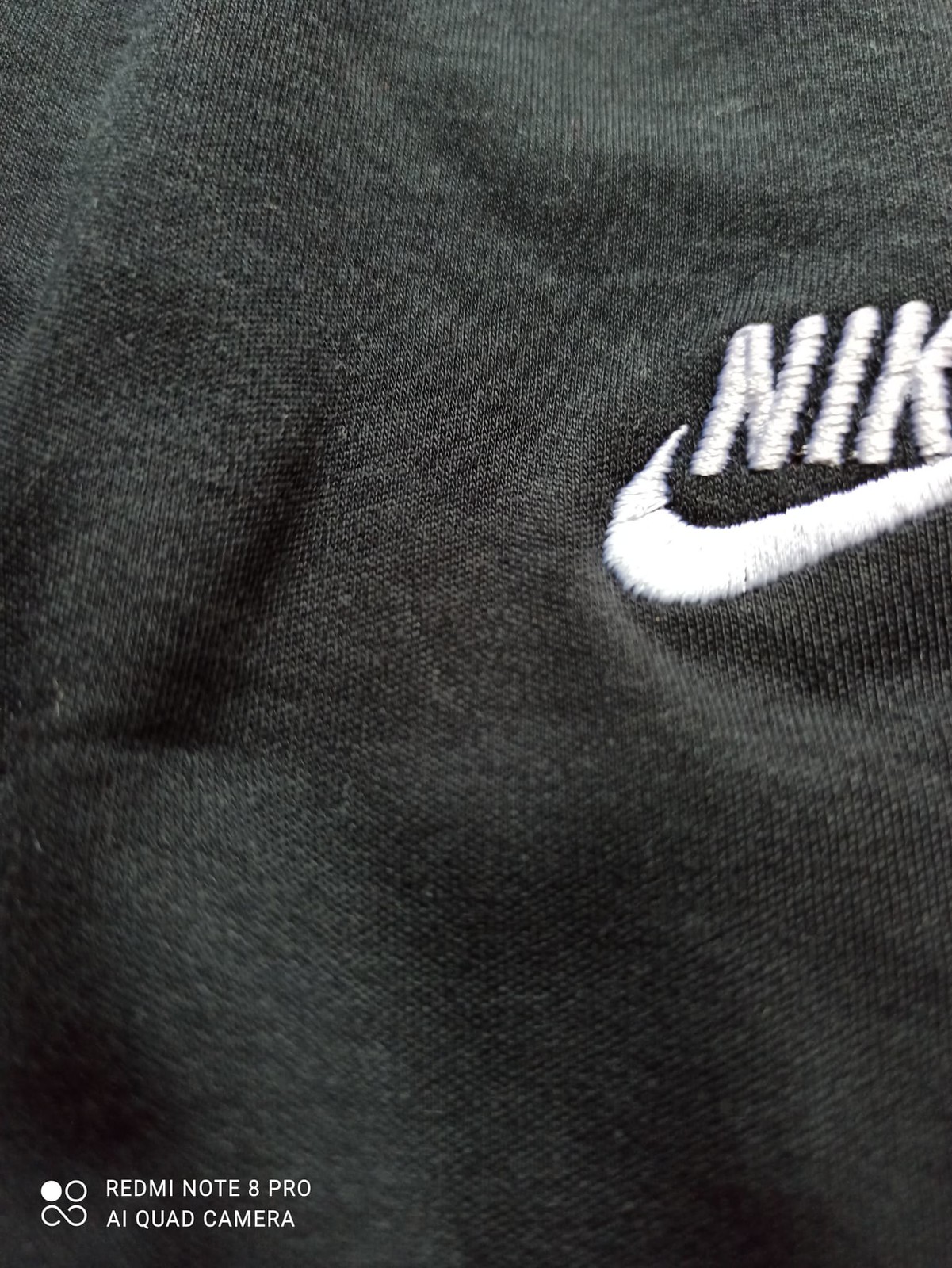This image features a close-up view of a black fabric, showcasing intricate details and textures. The material has visible wrinkles throughout, adding depth and highlighting the fabric's texture. Positioned in the top right corner is a partial view of the Nike logo, with the letters "NIK" in bold white embroidery, though the last character is cut off from the frame. Below the partially visible text, the iconic white Nike checkmark is also embroidered, reinforcing the brand's identity. In the bottom left corner, there's a faint watermark featuring a white circle with an empty circle inside and an infinity symbol beneath it. Accompanying this symbol are the words "Redmi Note 8 Pro" and "AI quad camera," indicating the device used to capture the image.